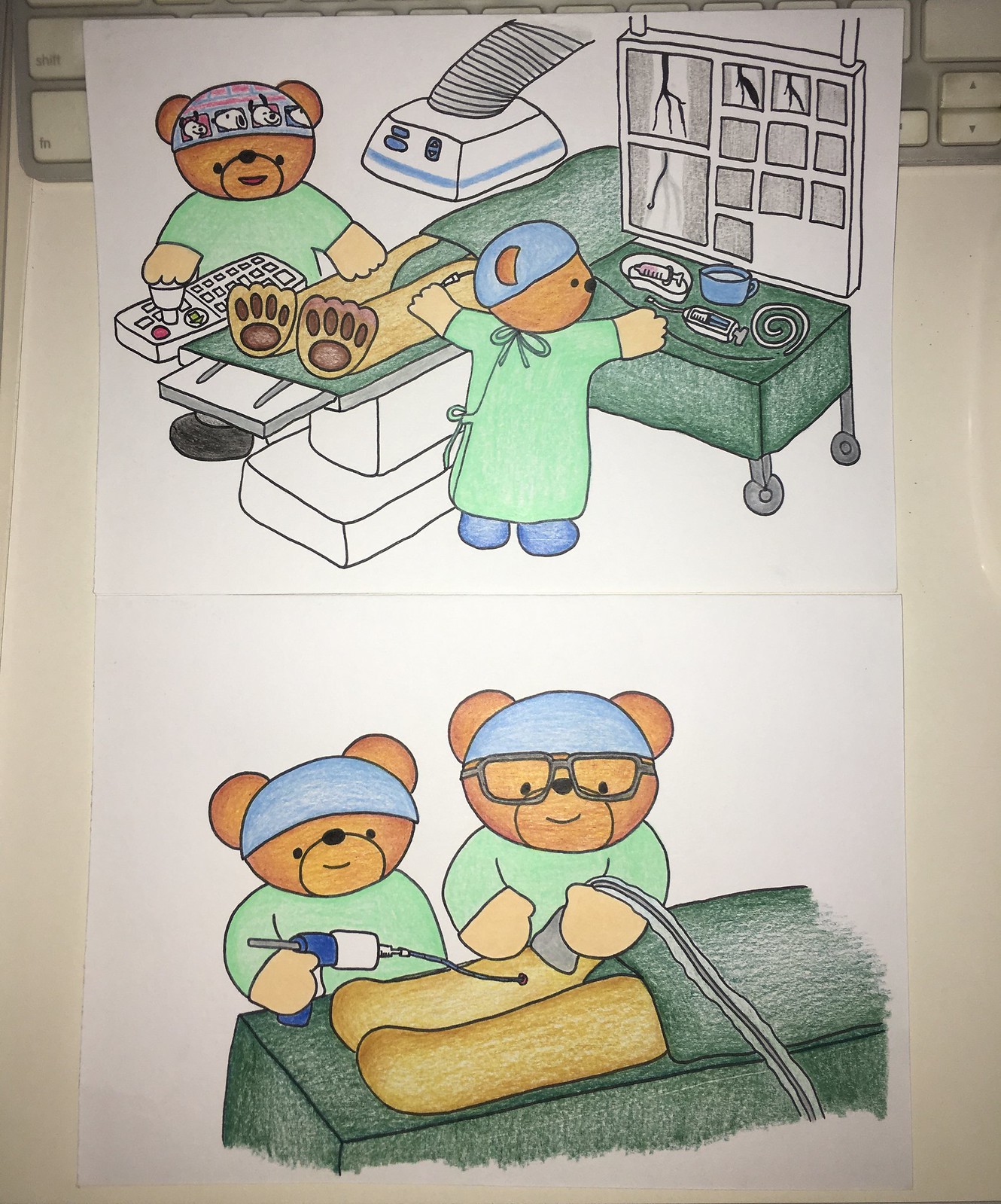The image features two intricately drawn illustrations, created with pen and colored pencils, on separate sheets of paper stacked upon each other. The top drawing rests on a keyboard, providing a casual workspace backdrop.

In the first illustration, two teddy bears are depicted performing surgery on a cream-colored patient bear, identifiable by its claws and paws. The bear on the left, adorned with a Snoopy-patterned hair net, operates from behind a console that includes a keyboard and joystick, suggesting the use of surgical robotics. This bear is brown and dressed in green surgical scrubs. 

On the right, another teddy bear in green scrubs and a blue hair net focuses on a detailed procedure. This bear manipulates a device over the patient and examines an adjacent screen displaying multiple x-rays. A large x-ray machine looms above the patient, illustrating the device's function. The operating table below is cluttered with various surgical tools, including a syringe.

The second illustration beneath depicts a similar surgical scene but with slight variations. Here, two teddy bears, also brown and clad in green scrubs with blue hair nets, appear to engage in a surgical procedure on the patient. One bear wears glasses and operates a vacuum-like device, while the other handles a syringe or gun connected by a tube to a wound on the patient's leg, indicating a focused surgical intervention. The meticulous details in both drawings showcase a whimsical yet serious portrayal of teddy bears in a medical setting.